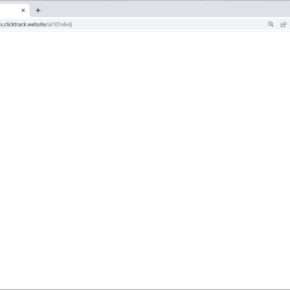The image captures a computer screen displaying a web browser. The background is predominantly white. At the top of the screen, there's an open browser tab, although it is quite blurry, making specific details hard to discern. There is visible black text within the tab, and an 'X' icon is in the upper left corner of the tab, indicating where you can close it. Beside this tab, there's a gray area featuring a '+' icon, used for opening a new tab.

The central portion of the screen is blank and white, suggesting an inactive or newly opened browser window. Toward the bottom, a faint horizontal gray line stretches from the left edge to the right edge of the screen. A similar faint gray line is also visible at the top.

In the top gray area, there appears to be another clickable item, but it is too blurry to identify, even upon zooming in. The overall composition suggests a minimalistic and clean browser interface, with the focus on the simplicity of open tabs and navigational elements.